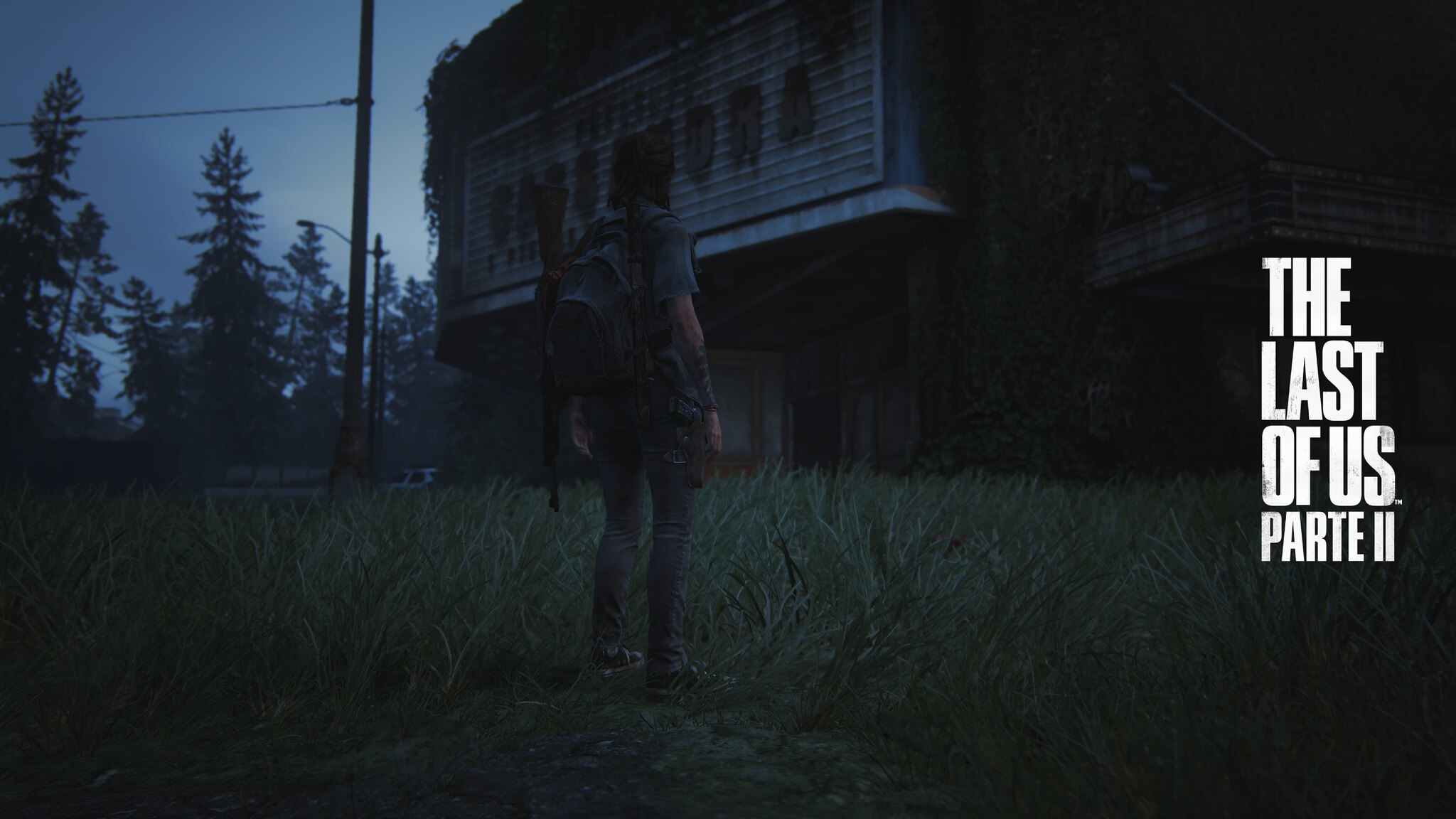This is a rectangular landscape image, nearly twice as wide as it is high, with a predominantly dark theme. In the center of the image, a man stands on a thick grassy field, with his back partially turned to the viewer and facing a large, dimly lit building. The man appears to be wearing tight jeans, a short-sleeved shirt, and a backpack, with long, dark hair flowing down his back. The image is very dark overall, with the lower 40% dominated by grass and shadow.

On the right side of the image, there is a multi-storied building that extends from the center to the far right edge. The building is difficult to detail due to the darkness, but it features a row of 7 or 8 windows across the top level, hinting at its layered structure. The man seems to be gazing upward at this building.

In the upper left corner of the image, tall, fur-like evergreen trees are silhouetted against a dark blue sky, though most of the sky and background remain shrouded in shadow. 

Overlaying the image, in white all-caps font, are four rows of text stating "THE LAST OF US" and below it, "PART II" (with "PART" written in uppercase letters and "II" in Roman numerals). These lines are stacked near the right side of the image, slightly left-justified.